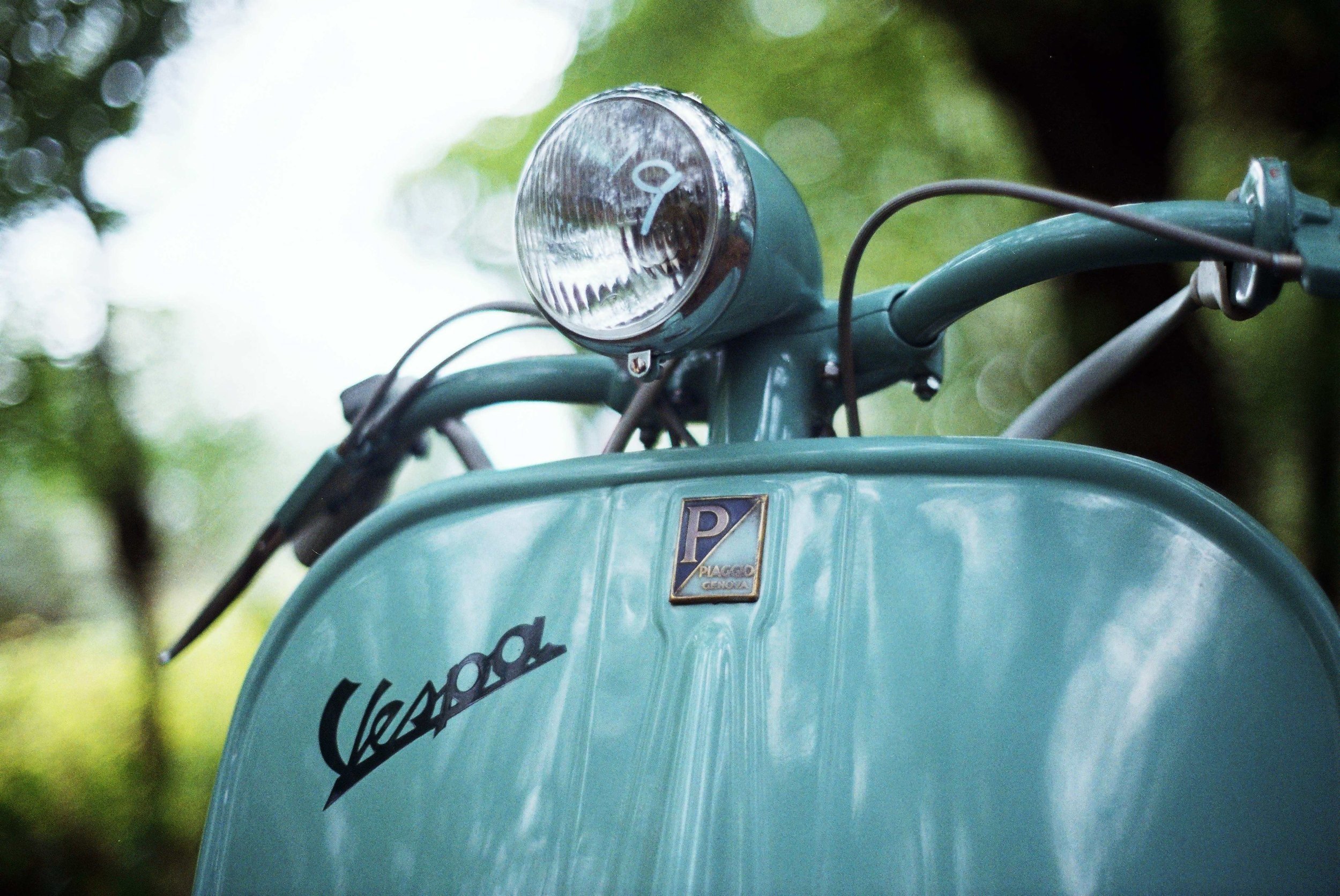This photograph captures the front section of a turquoise Vespa scooter, focusing on the upper part of its body, known as the shield, which functions as a windbreaker for the rider. The headlight, positioned in the top center, is encased in a chrome rim and appears slightly domed like a bulb. The distinctive Vespa logo, featuring an inclined script font in a black shade, is prominently displayed on the lower left of the shield. Below the logo, there's a rectangular metal badge with a "P" symbol and smaller text.

The handlebars extend from the shield, framing the headlight. A notable feature is a handwritten number "9" with a white marker on the headlight. The background blurs into a blend of green vegetation and overexposed sky, indicating a sunny day with trees or foliage, though these elements remain out of focus to emphasize the scooter.